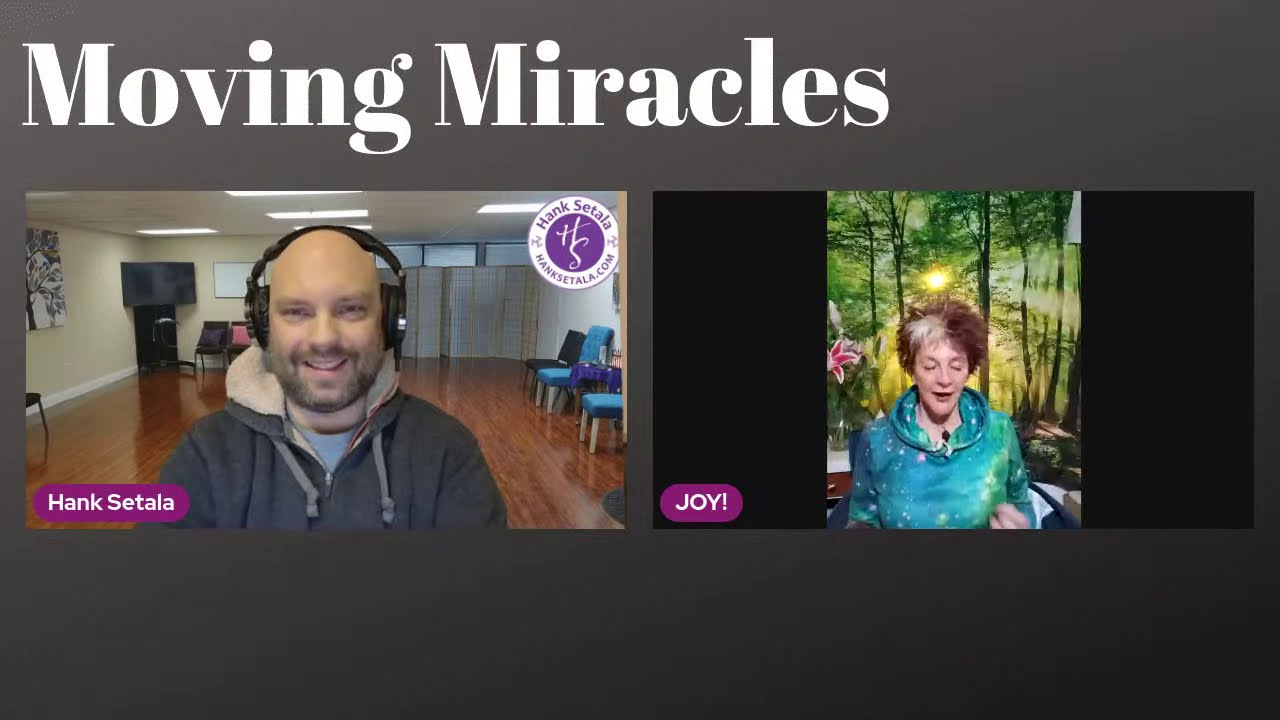The image titled "Moving Miracles" features a dark gray background with the title written in serif white font at the top, where the M in "Moving" and the M in "Miracles" are capitalized. Below the title, the image is split into two side-by-side segments. 

On the left, the picture shows a man named Hank Sitala, identified by the text in a purple pill-shaped bubble with white font in the bottom left corner. Hank is a white man, likely in his late 30s or early 40s, with a mustache and a beard of dark grayish-brown color. He is bald and is wearing black over-the-ear headphones. He sports a gray coat with a hat that has a zip opening, slightly smiling while staring straight ahead. Behind him, there's a TV mounted in the corner where two walls meet, a shiny brown wooden floor, and blue chairs set against a white wall. At the top right of Hank's picture, there's a logo with a circle bearing the initials "H & S" and the words HankSitala.com in the surrounding ring.

On the right side of the image is a picture of a woman named Joy whose name is in all capital letters with an exclamation point, also in a purple bubble with white text. Joy has short brown hair and is wearing a blue and green dress with white spots. The background behind her features an image of a forest with sunlight streaming through the trees.